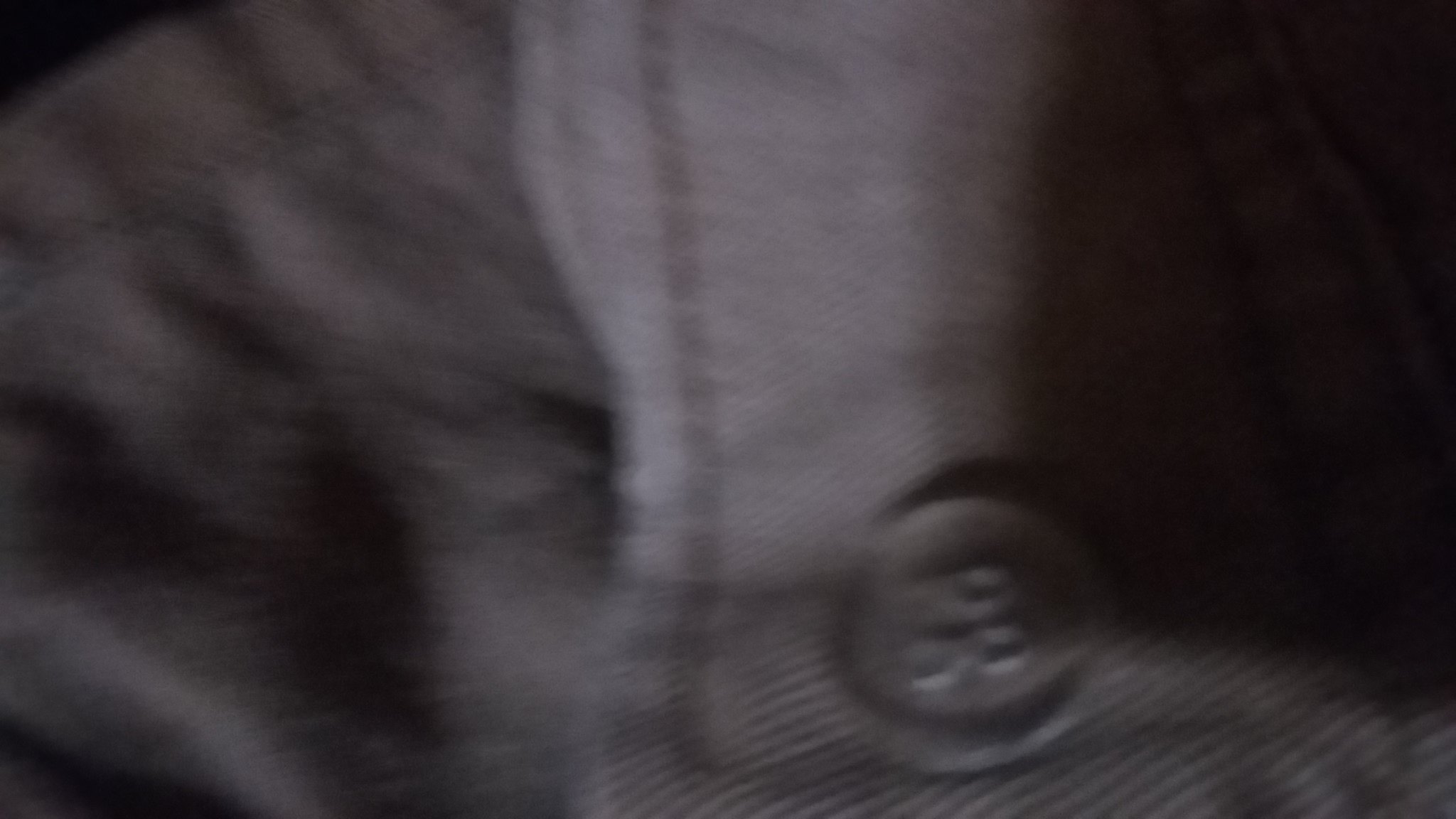The image depicts a close-up view of a mostly black fabric shirt. Prominently featuring a vertical stitch line running up and down the shirt, it intersects with a horizontal stitch line across the top. The fabric displays natural folds and dark shadowing, suggesting a soft texture. On the right side of the shirt, there is a button with the letters "PR" embossed on it, accompanied by concentrated black shadowing. Additionally, subtle lines traverse the shirt, contributing to its intricate design. The lighting in the image creates a gradient effect, with the top portion being illuminated to a light gray and progressively darkening to a deeper gray towards the bottom, with more pronounced shadowing on the top right. The overall image is slightly out of focus, adding a delicate, almost ethereal quality to the visual.